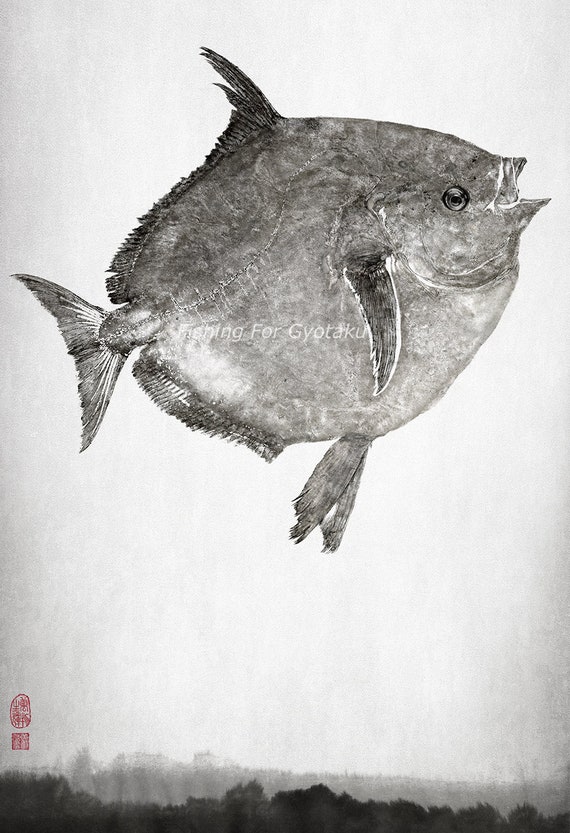A black and white image captures a highly detailed, almost photorealistic drawing of a fish, possibly a flounder, floating against a seemingly surreal backdrop. The fish is flat and round, facing the right with its open beak-like mouth. It has a prominent dark dorsal fin on its back and a similarly dark side fin near its eye, complemented by two lighter-colored fins on its underside. The tail is small, positioned on the left side of the image, contrasting slightly in shade. The background features what appear to be mountains or a foggy landscape towards the bottom edge, adding a mystical feel. The scene is reminiscent of the fish flying in a sky that transitions from light at the top to darker shades near the bottom. There is a white text watermark across the fish’s body, partially legible as "4GYOTAKU," and a red symbol located in the bottom left corner of the picture.